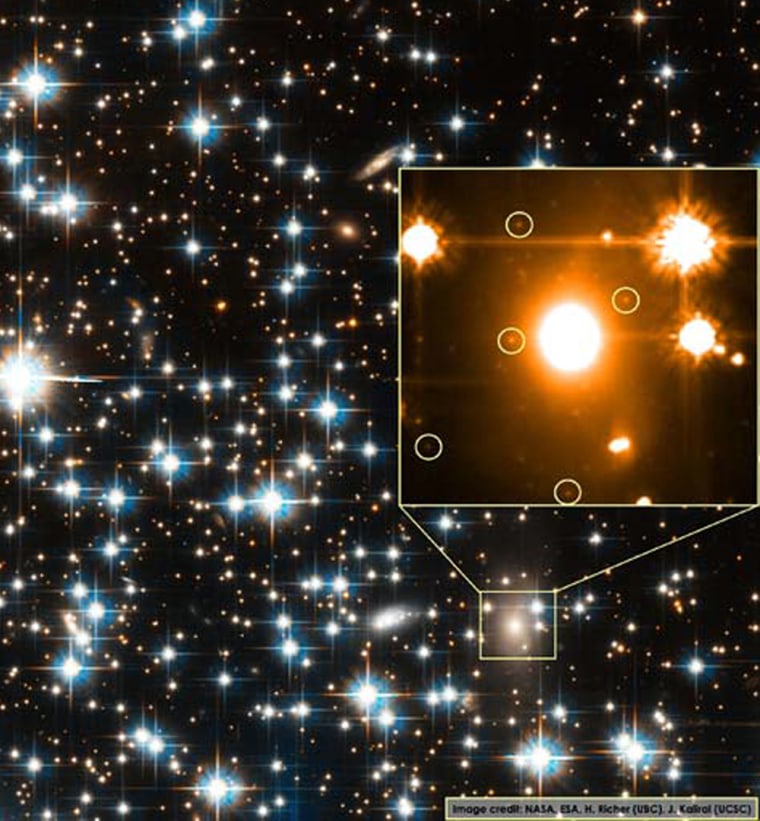This vertical image captures a star-filled night sky set against a deep black background. The sky is sprinkled with numerous white dots of varying sizes, mimicking stars—some are large and bright, while others are smaller and dimmer. The majority of these stars shine with a radiant, star-like quality, filling the entire frame with their luminescence.

There are also stars that exhibit different colors, including blue and orange hues. Two primary areas are emphasized: two stars have a distinct square around them, and a larger square to the right central part of the image displays a zoomed-in view of these stars. This close-up highlights stars of diverse shapes; some are perfectly round with clean edges, while others have jagged contours. Inside this zoom-in section, bright orange stars with smaller spots are also visible.

At the bottom right of the image, there is text within a small bordered box, too diminutive to decipher clearly. Additionally, there is a credit notation at the bottom, "Image credit: NASA, ISA, M. Eichner, Jay Capra," acknowledging the contributors to this stellar photograph.